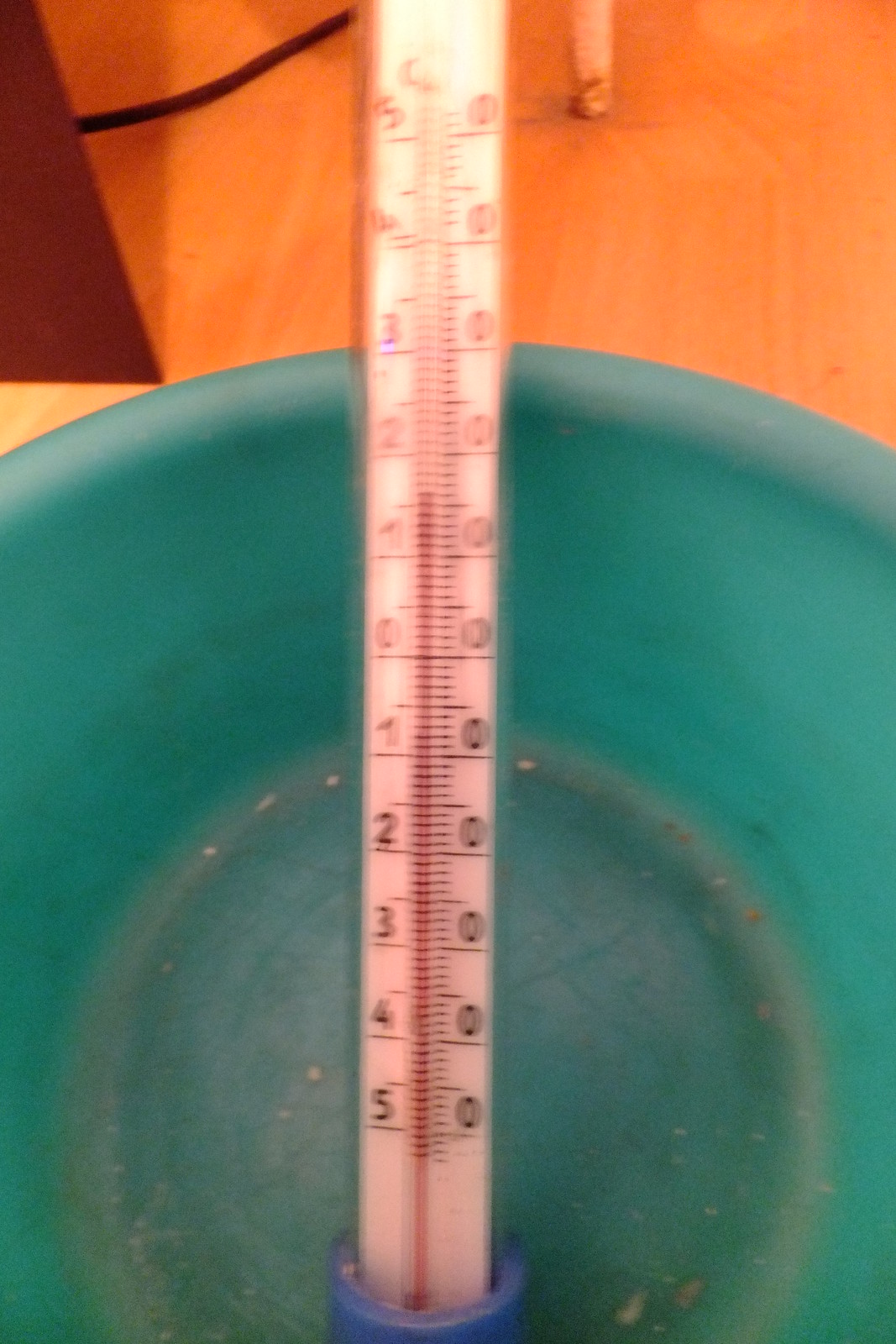The image is a color photograph presented in an upright or portrait orientation, resembling a vertical rectangle. It is slightly out of focus, giving a soft blur to the details but retaining enough clarity to identify objects. In the upper section of the photo, the background seems to feature elements such as a floor, the edge of a cabinet, and potentially a tabletop along with another cabinet edge. A black irregular line, possibly an electrical cord, snakes through this background.

Occupying the main lower two-thirds of the image is a blue-green, translucent plastic bowl that appears well-used and worn, with noticeable scratches on its surface. The bowl is empty except for minor residue, including a few white spots at the bottom.

Inside the bowl and extending from the bottom of the image to its cropped top is a measuring device that closely resembles a candy thermometer. This glass thermometer has a round appearance and contains a red mercury-like line indicating temperature. The increments on the left side of the thermometer scale range from 5 down to 0, and continue upwards from 1 to 5, while the right side displays only zeros. The red mercury line marks a reading of approximately 1.5 above the central zero. At the base of the thermometer lies a blue plastic case, partially cropped from view at the bottom of the image.